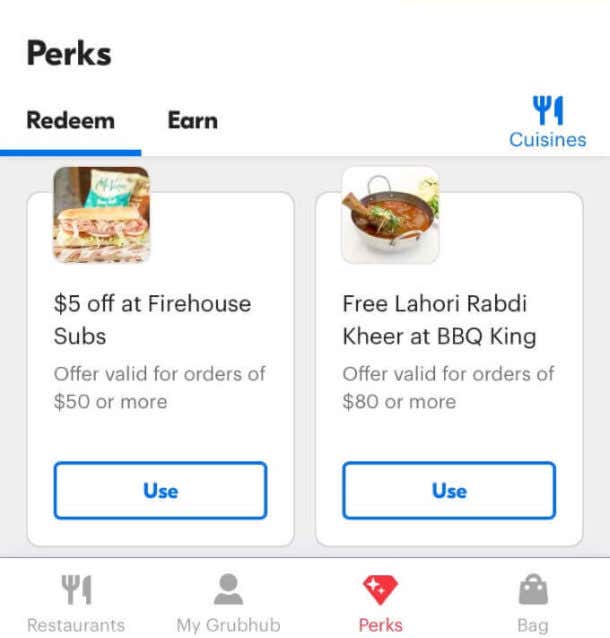The image is a square-shaped screenshot from the Grubhub app, showcasing the "Perks" section, prominently displayed in bold font in the upper left-hand corner. Below this title, there is a navigational row with three choices: "Redeem," "Earn," and an icon of a fork and knife with the label "Cuisines." The "Redeem" option is currently selected.

The main portion of the screenshot features two different food deals. The first deal includes an image of a sub sandwich accompanied by some chip bags. The text beneath this image reads: "$5 off at Firehouse Subs. Offer valid for orders of $50 or more." There is also a "Use" button provided to redeem this offer.

Adjacent to this is the second deal, which showcases a stainless steel pot with handles, filled with a reddish-colored soup or stew. The dish appears to contain some sort of meat or protein, garnished with vegetables on top. The text associated with this image states: "Free Lahori Rabdi Kheer at BBQ King. Offer valid for orders of $80 or more."

The bottom of the screenshot includes three navigation options: "Restaurants," "My Grubhub Perks," and "Bag," allowing users to easily access different sections of the app.